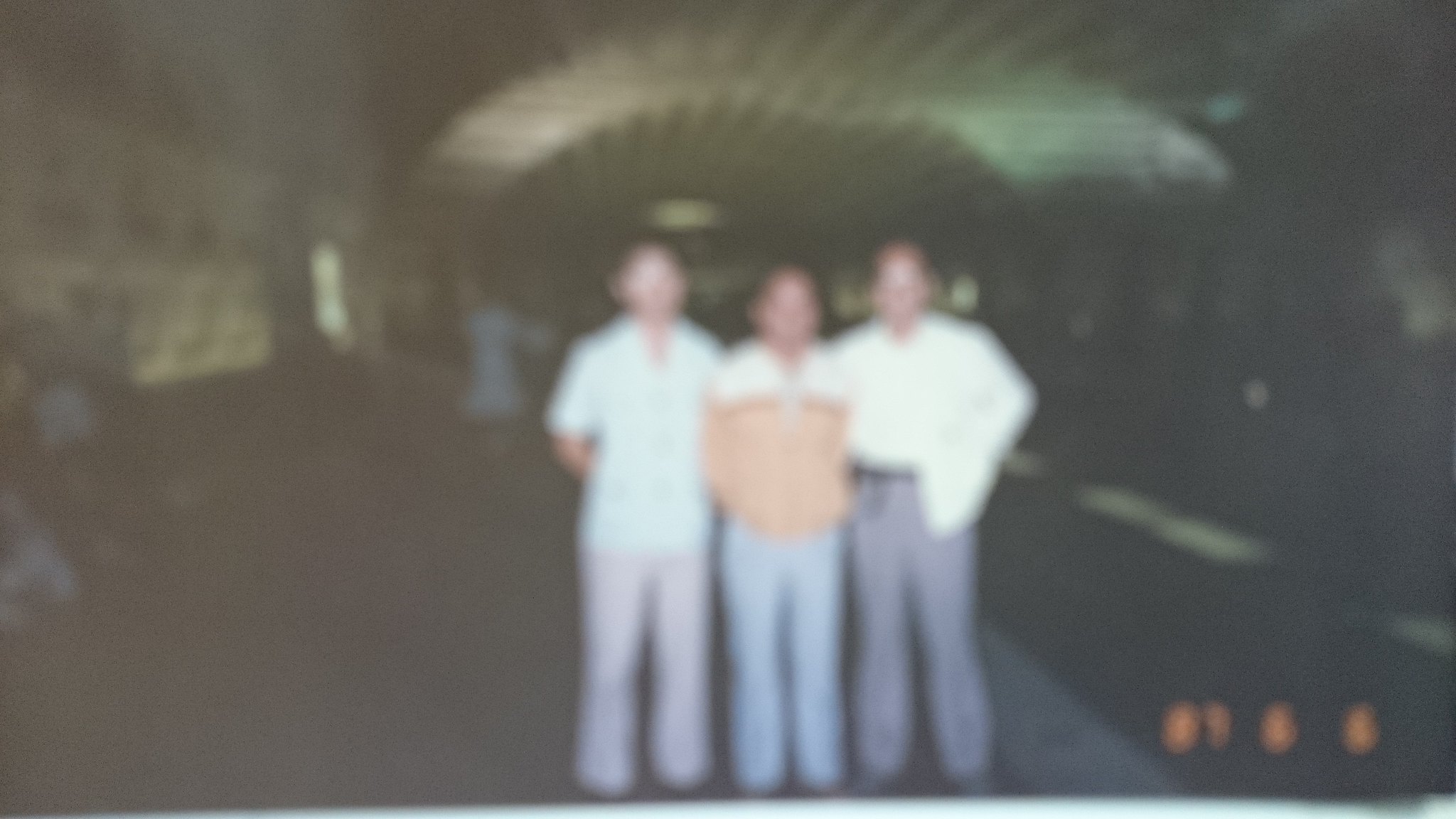This is a really old, dark, and blurry color photograph, likely from the 1960s or 70s, capturing three men standing together in the London Underground. The ambient lighting reveals an arched roof in the background, subtly illuminated, while the dark environment partially obscures the scene. At the bottom right, a faint orange date is visible but incomprehensible.

The three men, possibly of Southeast Asian descent, stand with their arms around each other. On the left, a man in a light blue short-sleeved shirt and gray flared pants, possibly bell-bottoms, poses with his hand behind his back. The man in the center is slightly shorter than the others and wears a distinctive orange T-shirt or jacket with a white top section, an orange stripe across the chest, and lighter orange lower sections, paired with light blue or gray pants. The man on the right sports a long-sleeved white shirt, part of a white jacket, and gray pants, with one hand in his jacket pocket and the other resting behind the central man. To the right of the photograph, you can also glimpse part of the subway track.